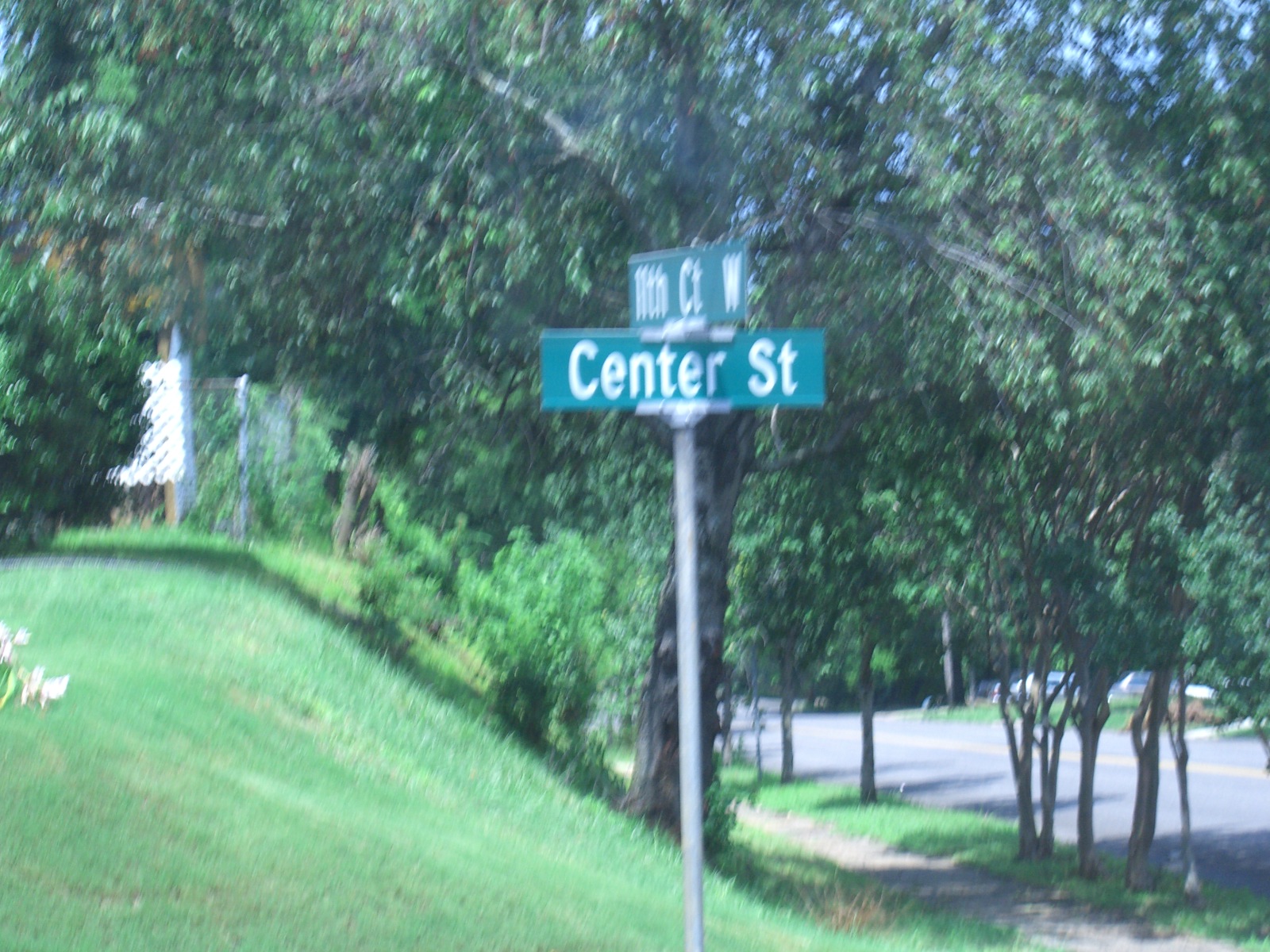The image depicts a typical suburban street sign in the United States, located at an intersection. The green street sign with white text indicates two streets: "Center St" (abbreviated as "CENTER ST") and "11th Court West" (abbreviated as "11TH CT W"). The streets intersect at right angles, evidenced by the perpendicular alignment of the signs atop a silver-gray pole extending from the ground.

In the background, a suburban street scene unfolds. While the image is not entirely clear, it reveals a sidewalk lined with trees, some cars in the distance, and a road marked with a central yellow line. Although no houses are visible, the scenery is characterized by dense greenery, including trees and a hill behind the sign. Fencing is also visible in the backdrop, contributing to the suburban ambiance. The overall palette of the image is dominated by green, thanks to the lush tree cover and the hill behind the street sign.